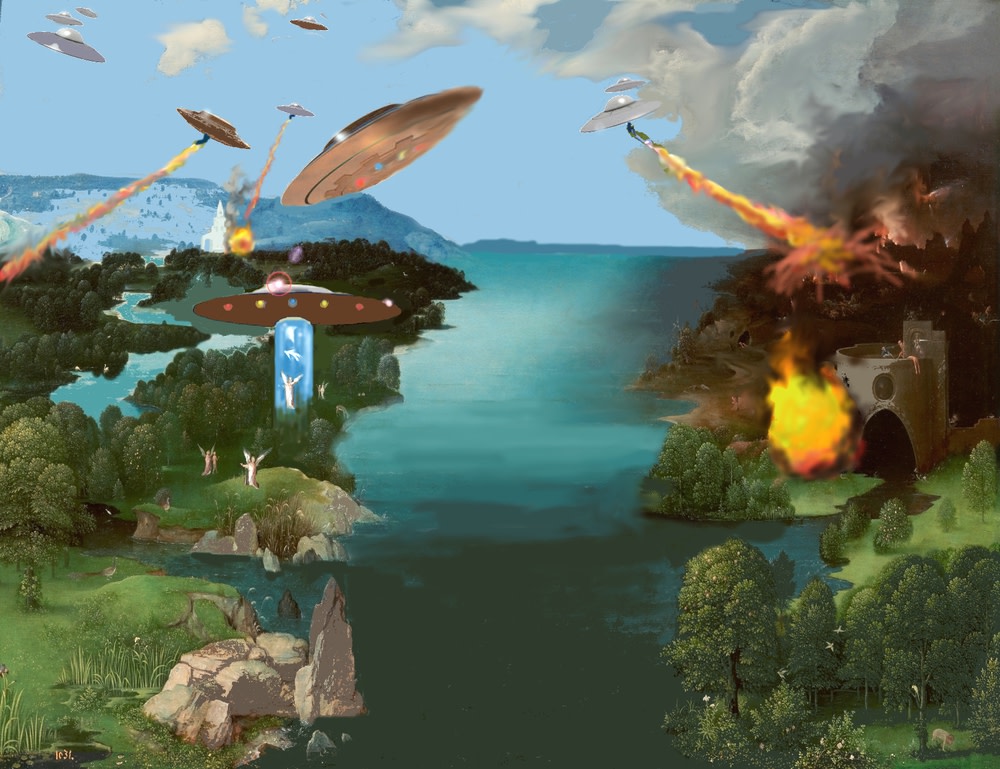The painting is a striking blend of vibrant, surreal, and somewhat realistic elements reminiscent of Dali or Bosch. Dominated by shades of blue, the centerpiece is a dark blue river or body of water that draws the viewer's eye toward the center. On either side of the water, lush, dark green landscapes teem with trees, grassy areas, and occasional rocks. The sky above is a light blue expanse dotted with fluffy white clouds.

The surreal aspect of the painting is highlighted by the presence of numerous flying saucers, nine in total, engaging in what seems to be a chaotic battle. Some saucers are discharging weapons with trails of fire, smoke, and explosions evident in the scene, particularly targeting and partially destroying a gray castle on the right side of the image. One saucer on the left features a tube-like beam pulling a person or angelic figure upwards. Scattered among the saucers are faint, small, white-winged beings.

Further into the background, you can make out a distant white castle or church, nestled behind more land and trees. Above the tumultuous landscape and amidst the chaos in the sky, the surreal battle-filled scene gives a striking contrast to the serene, pastoral image of the land below.